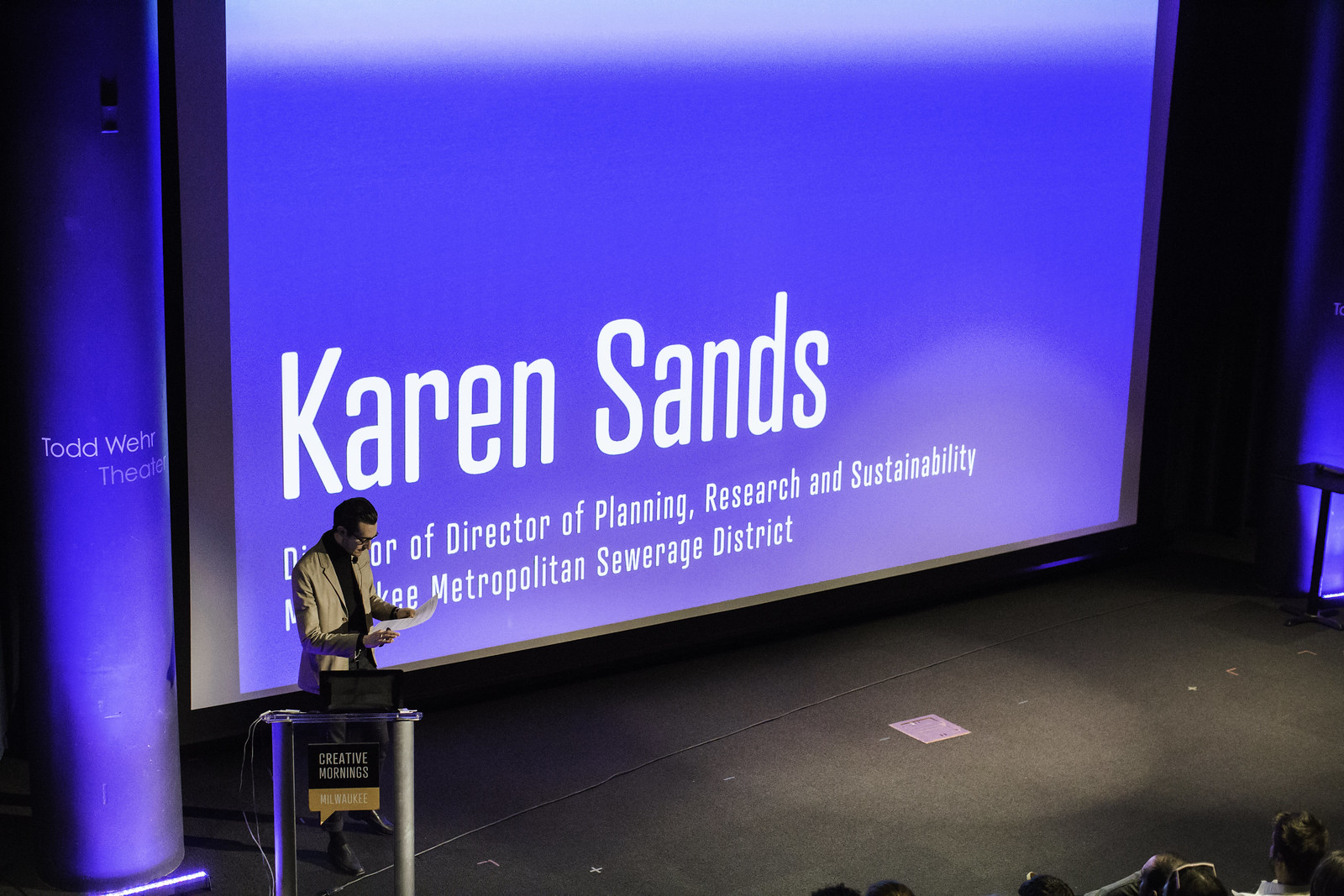This photograph captures a speaker at a conference held at the Todd Wehr Theater. The man, dressed in a white suit with a black undershirt and sporting short black hair, stands on a stage behind a small podium with a laptop. Behind him, a large projector screen displays a slide reading "Karen Sands, Director of Planning, Research, and Sustainability, Milwaukee Metropolitan Sewerage District," indicating a presentation about a new sewage project. In the lower right corner of the image, the heads of audience members can be seen. The podium features a sign with "Creative Mornings" in white text on a black and orange background. The man appears to either be reading or presenting information, though it's unclear from the image alone.